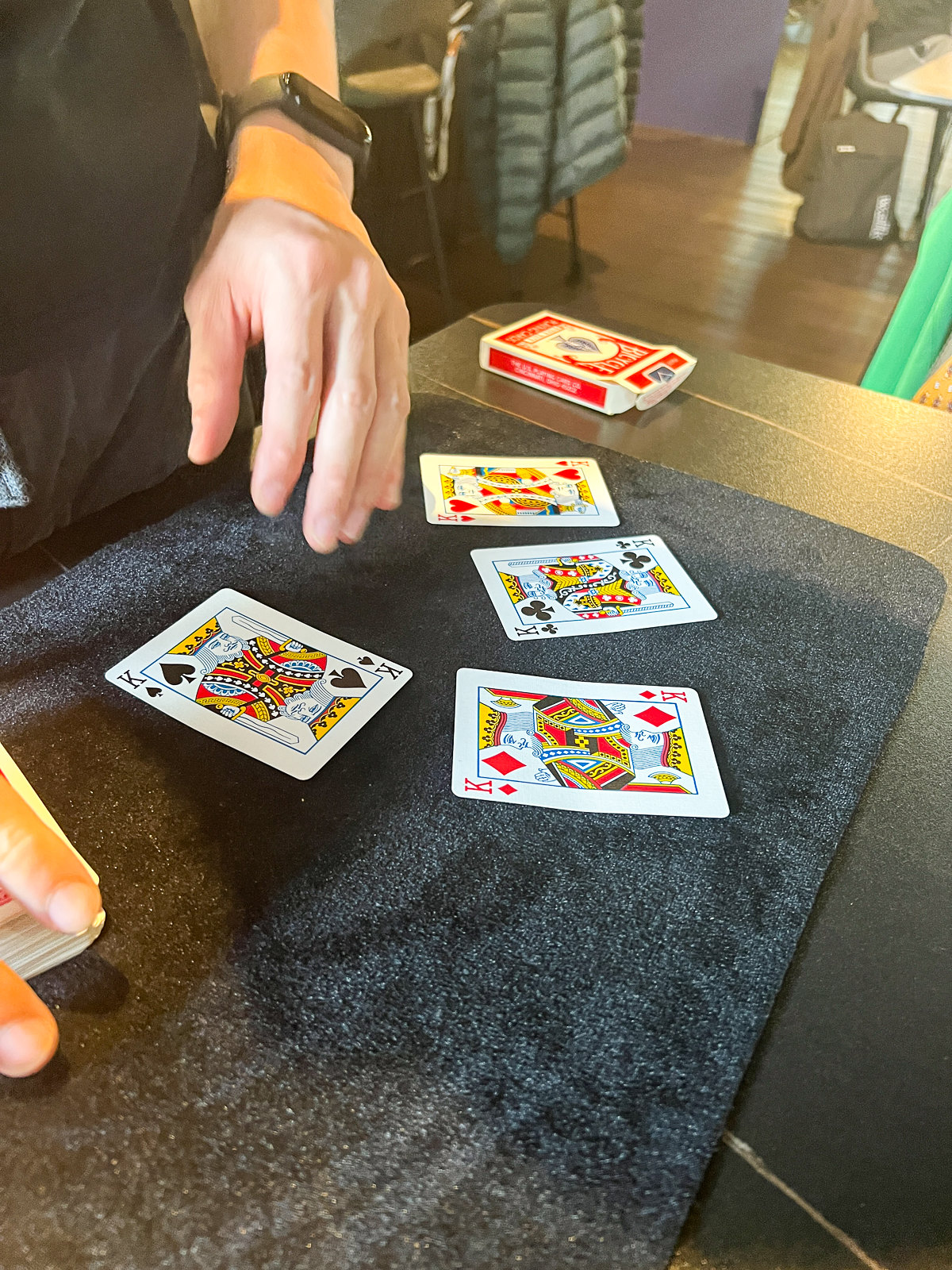In this overhead image, we observe a magician deftly manipulating a deck of playing cards atop a mat with a dense, star-galaxy design. The perspective reveals the magician's setup on a rectangular table, with the far end of the table visible at the top center of the image where a red and white deck of cards lies empty. This suggests the deck is currently held under the magician's fingers on the left side of the screen.

The magician, who has lighter skin and wears a square black watch on his right wrist, strategically displays four cards on his intricate mat. These cards, featuring the four kings, are meticulously arranged in a square pattern closest to the magician. The King of Spades is positioned almost perpendicular to the observer, orientated vertically towards the magician. Above it and to the right lies the King of Diamonds. The King of Clubs is situated behind the King of Diamonds, to the left from our view, while the King of Hearts rests closer to the magician, slightly to the left of the King of Clubs.

In the background, six cushioned chairs are stacked, partially covered by a coat, indicating that the setting may be in a hall, possibly during a wedding or reception. Another chair with a coat draped over it is also visible to the right. The precise arrangement of the cards and the formal setting contribute to the intriguing and professional atmosphere surrounding the magician's performance.